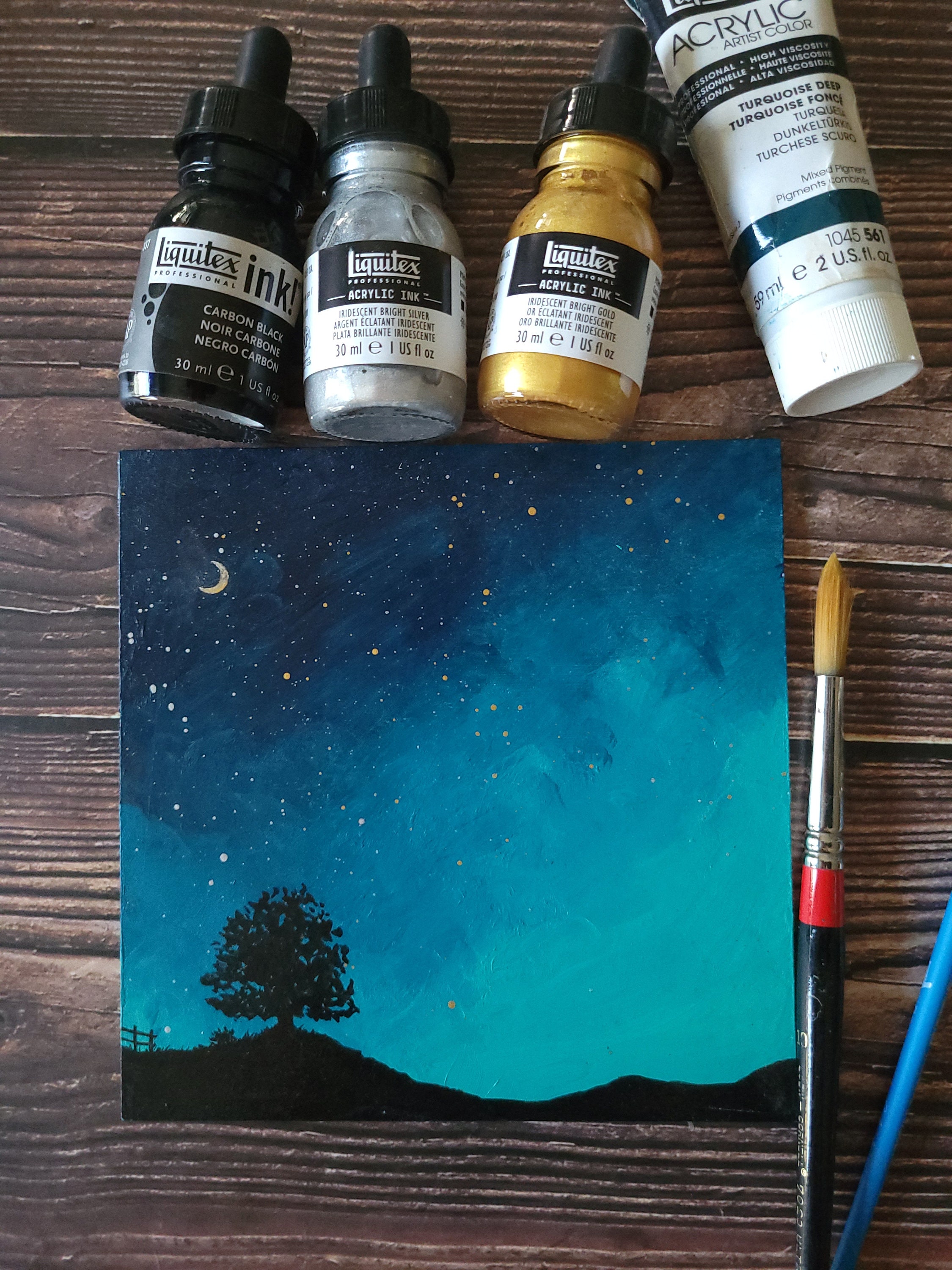The image features a small, square painting resting on a wooden table that showcases the natural color and texture of the wood. The painting, approximately the size of two iPhones put together, depicts a nighttime scene with a silhouette of a hillside and a single tree on the left. In the lower foreground, there's a hint of grass and a fence. The sky, which is predominantly blue, shifts from a lighter blue on the horizon to a darker shade as it ascends. A crescent moon is positioned in the upper left corner, accompanied by small dots representing stars. Above the painting are three glass bottles of acrylic ink in black, silver, and what appears to be gold. A tube of deep turquoise acrylic paint lies on the far right. Two neatly washed paintbrushes rest in the bottom right corner. The overall serene night scene in the painting evokes a landscape reminiscent of the 1950s movie "Invaders from Mars."